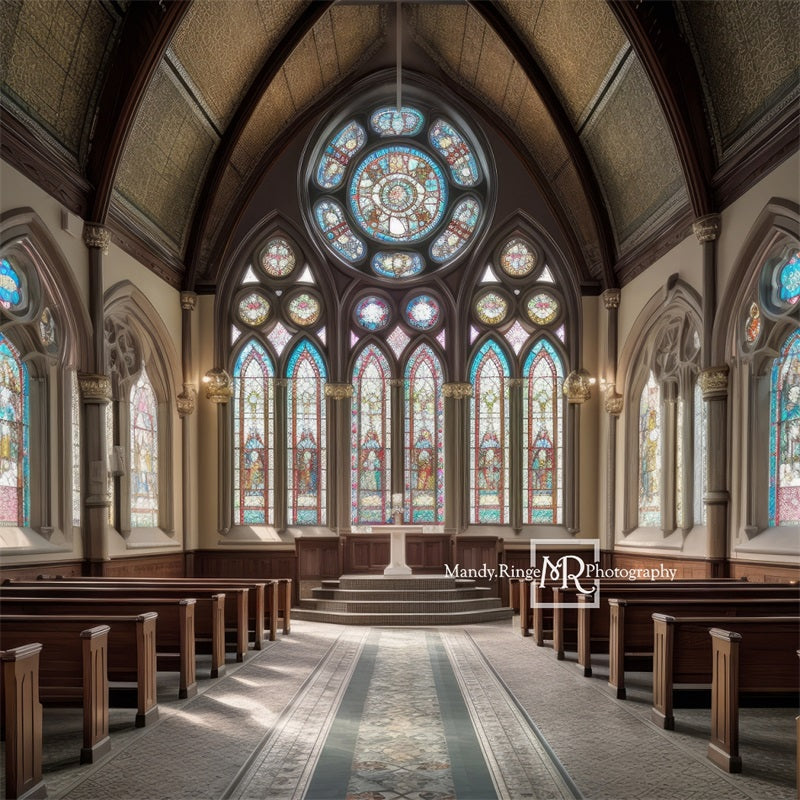The photograph captures the interior of an old church cathedral, highlighted by the watermark "Mandy Ridge MR Photography" at the bottom right. The spacious Gothic-styled church features numerous stained glass windows depicting various saints, adorning the left, right, and back walls. Prominently, a large circular stained glass window crowns the top of the back wall, beneath which three sizeable stained glass panels are displayed. An aisle runs down the middle, bordered by brown wooden pews on either side, leading to four steps ascending to a small white altar. The flooring is a plain flat surface, covered by a gray carpet with intricate designs. The walls are brown at the bottom and beige at the top, and the ceiling has a wooden brown hue. The structure of the church's front features a smaller arch followed by a larger arch, adding to its architectural grandeur. The photograph, void of people, exemplifies traditional edgings and classic ecclesiastical design elements.